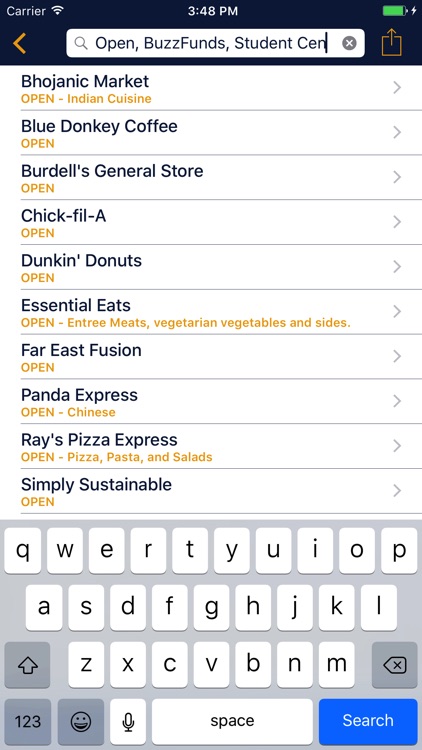In the image, a smartphone screen is prominently displayed, showcasing a list of various local businesses and eateries. The screen features names such as "Bohanic Market," "Blue Donkey Coffee," "Bordel's General Store," "Chick-fil-A," "Dunkin' Donuts," "Essential Eats," "Far East Fusion," "Panda Express," "Ray's Pizza Express," and "Simply Sustainable." Each entry provides information on whether the establishment is open, indicated in yellow, along with details about the type of cuisine offered, such as Indian cuisine for some entries. An arrow icon accompanies each listing, suggesting there is more information available. 

At the bottom of the screen is the smartphone's touchpad, which includes standard features like the gray background, square-like keys with black lettering, a blue "search" button, a white "space" button, and an emoji button, among others. This section of the screen indicates that the device is ready for text input.